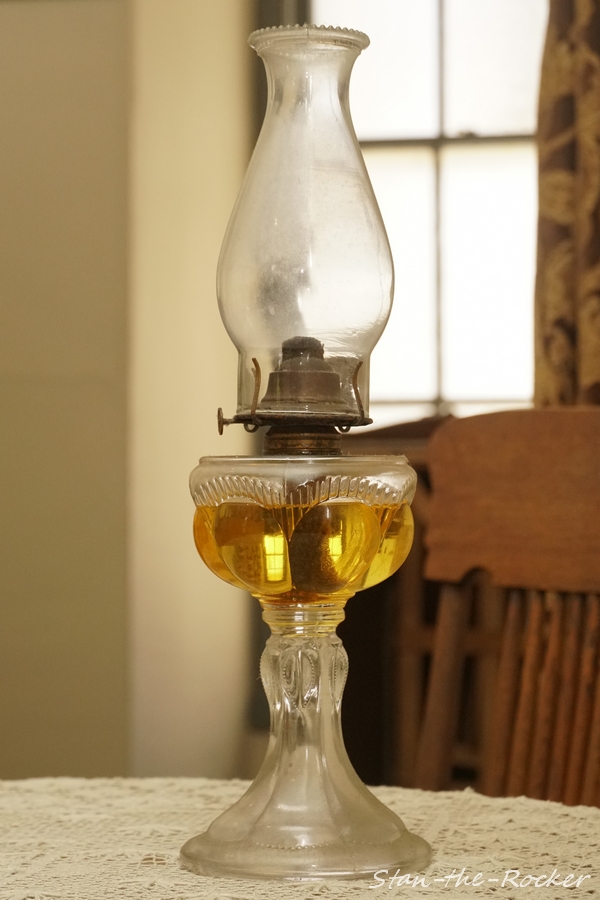The photograph captures an old-fashioned oil lamp made of translucent, foggy glass. The lamp, which stands on a table adorned with an intricate white doily or lace tablecloth, features a base shaped like a goblet, partially filled with yellowish oil. The wick is visible within the glass, leading up to a brass or possibly copper mechanical part that includes a small wheel for adjusting the wick's height. Topping the lamp is another glass piece designed to shield the flame. The setting is indoors, potentially within a kitchen or dining room, illuminated by light filtering through multi-paneled windows framed by flowered drapes. A wooden chair is visible in the background to the right. The photograph also contains a subtle watermark in the bottom right corner, reading "Stan the Rocker." The overall ambiance suggests a rustic and nostalgic scene.